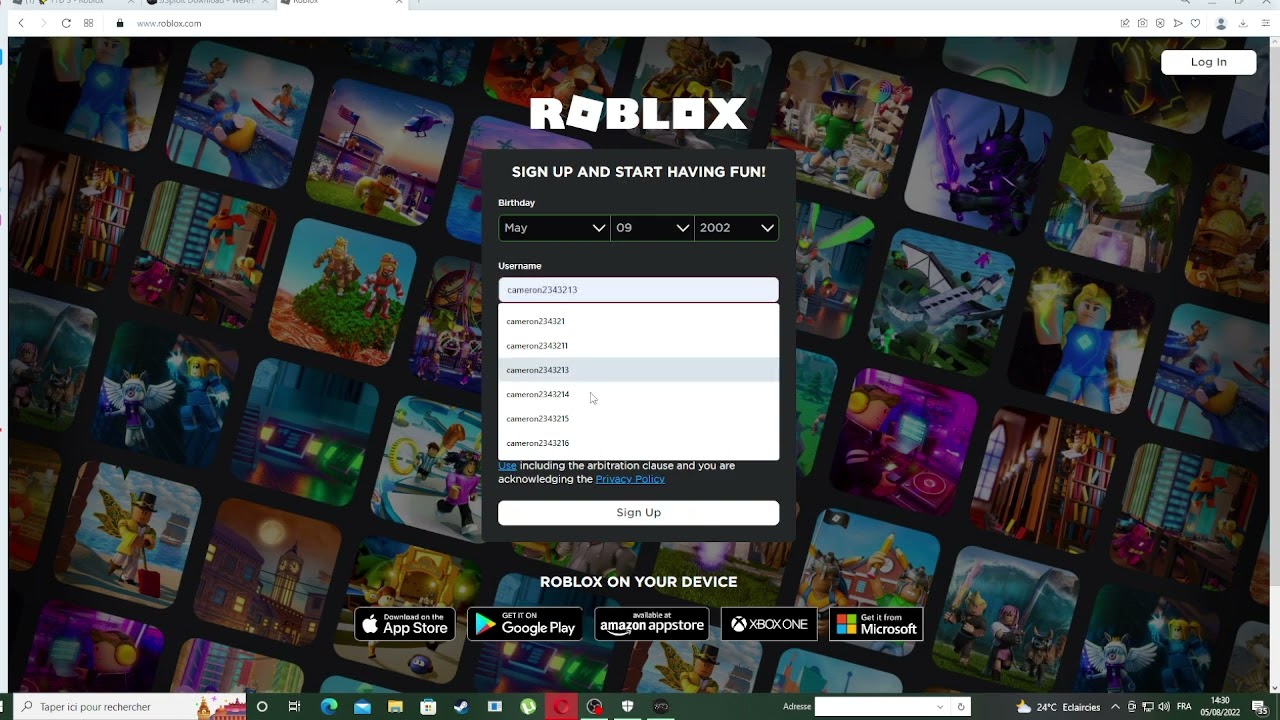The image showcases a desktop computer or laptop screen, with the web browser open to the Roblox website. At the top, the browser UI is visible, although slightly cut off, revealing three open tabs and the standard window controls. The URL bar distinctly displays "roblox.com." Dominating the screen, the iconic Roblox logo in stylized font is prominently positioned at the top.

Below the logo, there's a welcoming window encouraging users to "sign up and start having fun." This section exhibits a birthday field, populated with the date May 9th, 2002. There's a drop-down menu for selecting a username and a prominent sign-up button beneath it. Additionally, a section labeled "Roblox on your device" is present, featuring buttons for downloading the game from various platforms including the Apple App Store, Google Play, Amazon App Store, Xbox One, and Microsoft Store.

At the bottom of the screen, the Windows taskbar is visible, adorned with multiple pinned applications, a search bar, and the start menu button — all characteristic of a Windows operating system. The entire image is captured in a widescreen landscape format, presenting a comprehensive view of the setup.